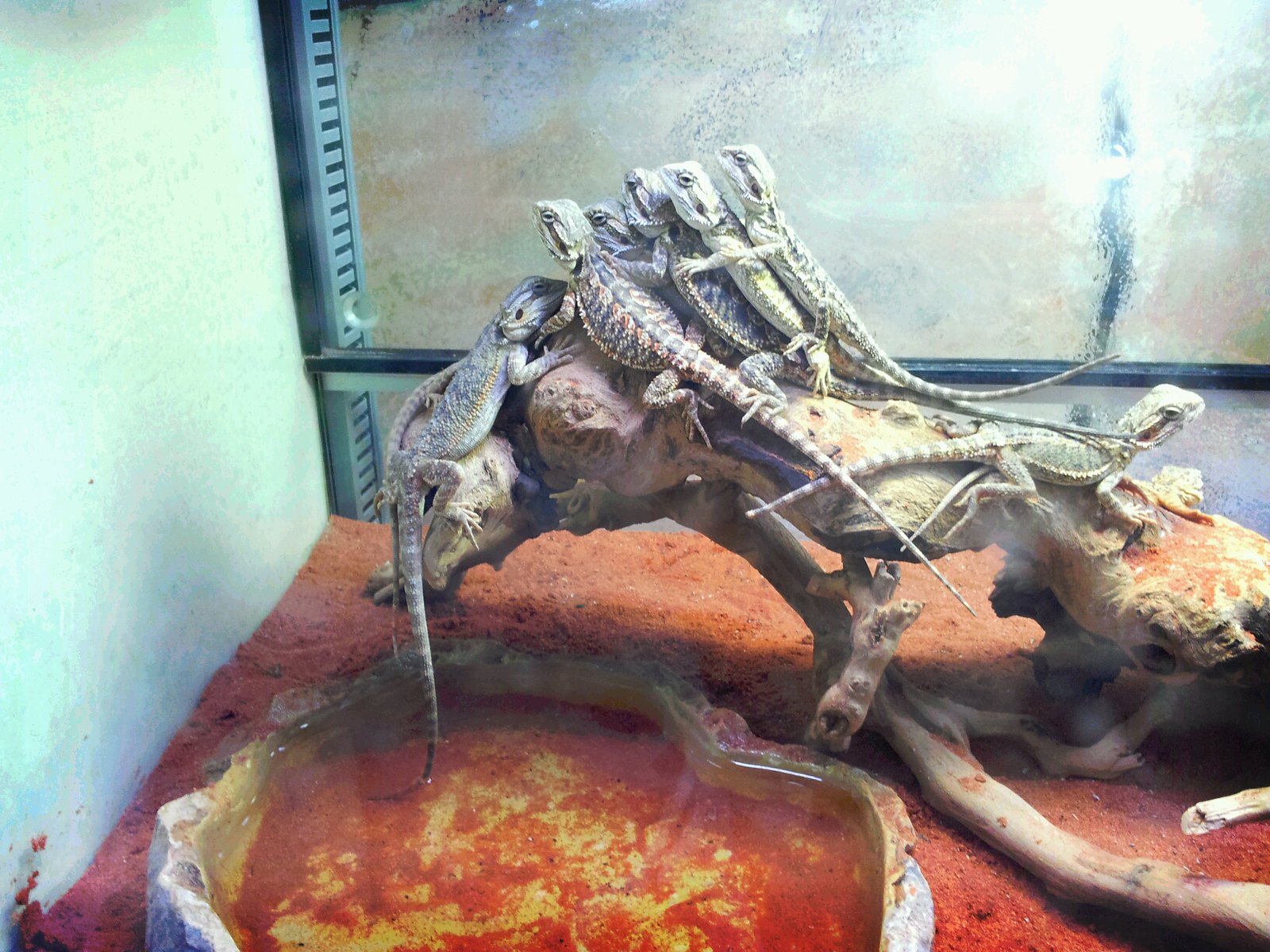This photograph showcases a terrarium housing several reptiles, likely bearded dragons or young iguanas. The terrarium's base is a vibrant mix of red clay dirt and orange sand. Positioned at the bottom left is a shallow, rock-shaped water bowl, containing a mix of water and red sand. At the center, a large piece of driftwood extends upward, providing a perch for the lizards. Four of the lizards are stacked atop one another on the driftwood, with their front legs touching the one in front. They feature a black and brown pattern down their bodies and long, thin tails. These lizards collectively face one on the left side of the driftwood, which gazes back at them. The enclosure is framed by foggy glass with a slightly greenish, mossy covering, supported by visible metal poles. The background includes a white wall, tinged with green.